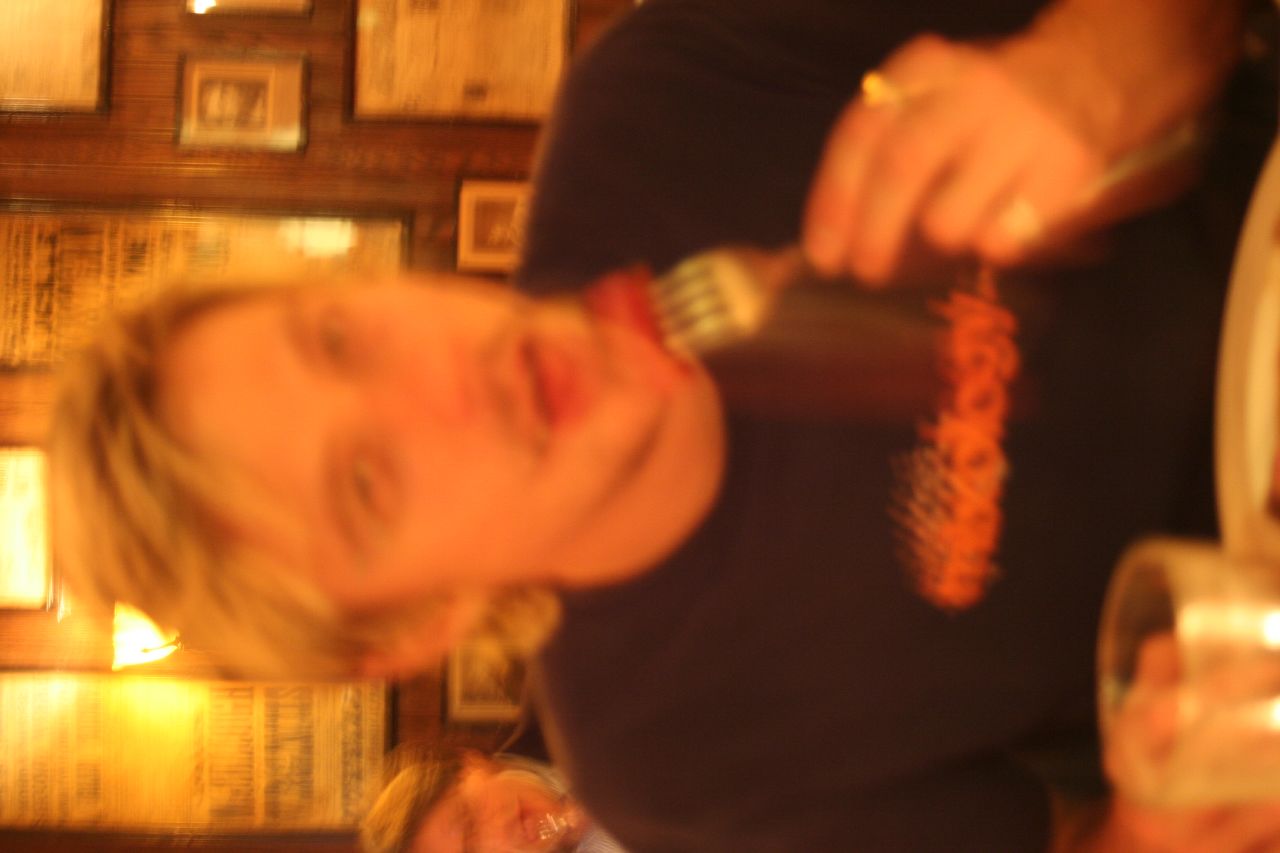A blurry photograph captures a young man in mid-meal at a restaurant. He appears to be Caucasian, with blonde hair revealing dark roots, a hint of a mustache, and noticeable dark circles under his eyes. The young man is holding a fork in his left hand, lifted to his mouth, and he wears rings on his index and possibly his little finger. Though the actual food on his plate isn't clear, the edge of the plate and a drinking glass are visible. In the background, another diner mirrors his action, holding a fork up to their mouth. The restaurant's decor is visible behind them, featuring wood-paneled walls adorned with numerous framed newspaper articles and photographs.